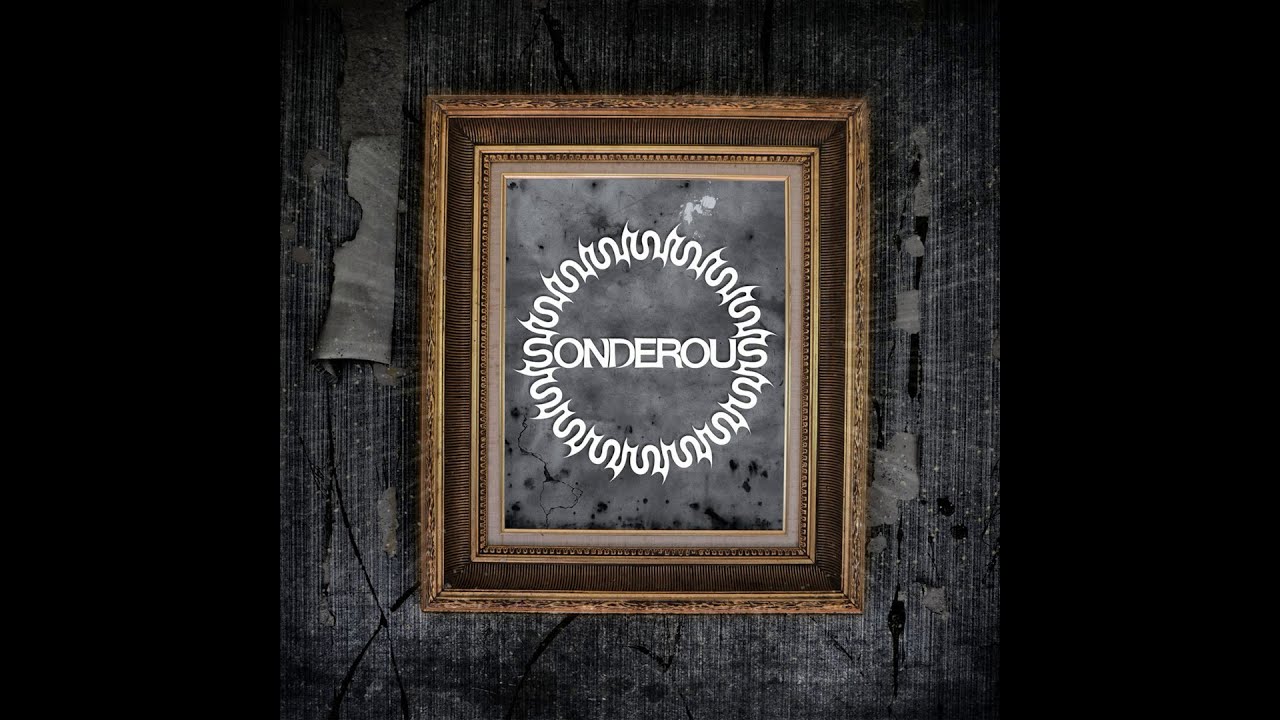This image depicts a framed portrait with an ornately decorated frame. The outer frame is detailed with a gold finish, transitioning into a brown, wood-like, or wicker material, before reverting back to gold with intricate detailing. A slim gold band lines the inner edge of the frame, encapsulating the actual image. The background of the portrait features a cracked, cement-like texture in shades of dark gray and black.

In the center of the image, a squiggly, circular pattern is formed by the letter 'S' repeated continuously, creating an almost snake-like effect. Within this circle, the word "Sondrous" is prominently displayed in white, capital letters. The area outside the frame resembles old, distressed wood in brown and gray hues, suggesting that the portrait might be laying on a wooden surface or perhaps against an old, wallpapered wall. The frame itself is finely detailed and medium to light in color, completing the overall ornate and slightly cryptic appearance of the piece.